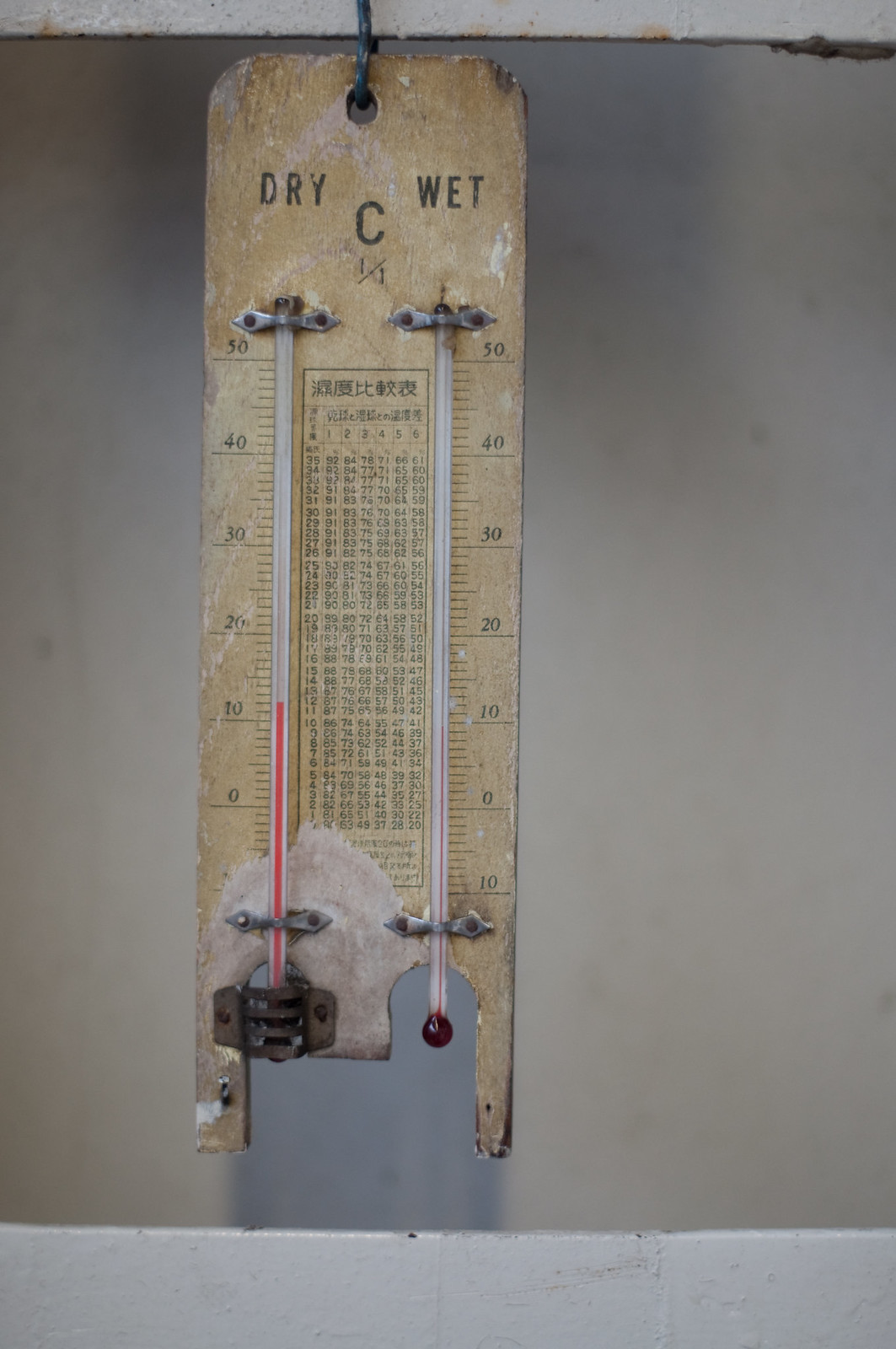The photograph captures an antique dry and wet bulb thermometer, hanging in portrait orientation. The device appears to be affixed to the interior or exterior rim of a window, hinted by the dark grout in the upper right corner connecting the rim, possibly a window frame. The rim itself is painted in a faded cream or light gray color with flecks of red. The window in the background is fogged up, suggesting high humidity, and it ranges from light to dark gray shades.

Central to the image, the thermometer is suspended from a small, dark black hook at the top center, with the thermometer’s base nearly reaching a painted light gray surface at the bottom, which has peeling paint hints. The thermometer appears quite old, with its wooden background painted a chipping light yellow. Sections of the wood reveal white, gray, and brown spots where the paint has eroded.

The thermometer features two distinct glass tubes filled with mercury. The left tube, labeled "dry," has a thicker mercury line indicating a temperature of 12 degrees Celsius. The right tube, labeled "wet," shows a thinner mercury line reaching up to 9 degrees Celsius. The readings are further segmented by silver bolts that hold the tubes in place; on the left, a more prominent and darker silver bolt is visible, while on the right, the bolt is missing, suggesting some wear and damage.

Between the two thermometers, there is a central chart marked with a combination of Celsius and possibly other units. The chart is structured into six columns, with numerical readings gradually decreasing from top to bottom. The top of the chart has a sequence of numbers in descending order, 35 through 1, with corresponding values listed in the six columns. These values start from 0 and incrementally increase up to around 61, adjusting every few lines. The exterior edges of the thermometers have additional scales graduated in decimals from 10 to 0, and back up to 10.

Overall, this intricate and worn piece serves as both a historical artifact and a weather-measuring instrument, showcasing the detailed craftsmanship of older scientific tools.